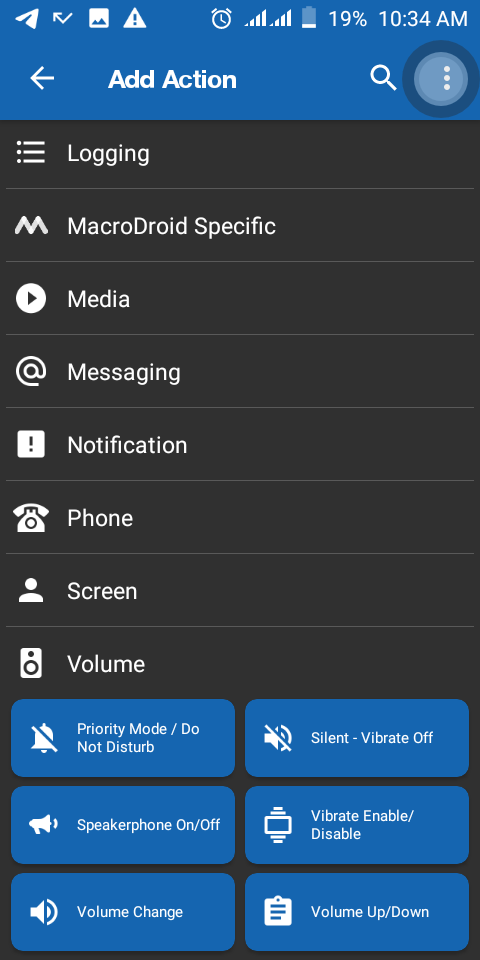The vertical image taken from a smartphone, predominantly features a user interface, likely from a task automation app. The top section of the image exhibits a midnight blue background with smartphone status icons displayed. On the upper left-hand corner, icons include a location icon, an arrow, a photo icon with a warning triangle, followed by the icons on the right: a clock, signal bar, possibly a string of notifications, battery life at 19%, and the time indicated as 10:34 a.m. 

Beneath this top row, on the left-hand side, there is a leftward-pointing arrow adjacent to the text "add action." To the right of this, there are a magnifying glass icon and a circle with three vertical dots, indicative of a menu for additional options. 

Below this header, the background transitions to a dull black, sectioning the content into a long rectangle with a thin white dividing line. Within this rectangle, a series of labels and categories are demarcated, each accompanied by its corresponding icon: Logging, MacroDroid Specific, Media, Messaging, Notification, Phone, Screen, and Volume.

At the bottom of the image, several rounded blue rectangular boxes are shown, each containing an icon and a label. These buttons likely represent various automation commands or settings: Priority Mode, Do Not Disturb, Speakerphone On/Off, Volume Change, Silent, Vibrate Off, Vibrate Enable/Disable, and Volume Up/Down.